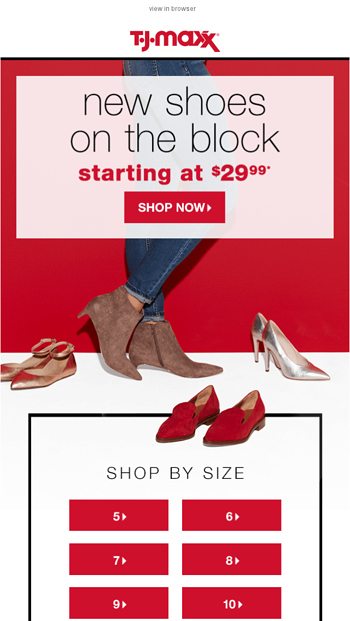This advertisement for TJ Maxx showcases their newest shoe collection. At the top, viewers are prompted to "View in Browser," followed by the bold TJ Maxx logo. The background is a stylish image of a person wearing a blue pair of jeans and a pair of leather or suede boots. To the left of the person are another pair of women's shoes, while to the right are a pair of elegant silver heels. In the forefront, striking red casual shoes take the spotlight. Overlaid on this fashionable imagery is the enticing text: "New Shoes on the Block, Starting at $29.99." A clear call to action invites shoppers to "Shop Now." At the bottom of the screen, customers can easily select their shoe size, with available options including sizes 5 through 10.